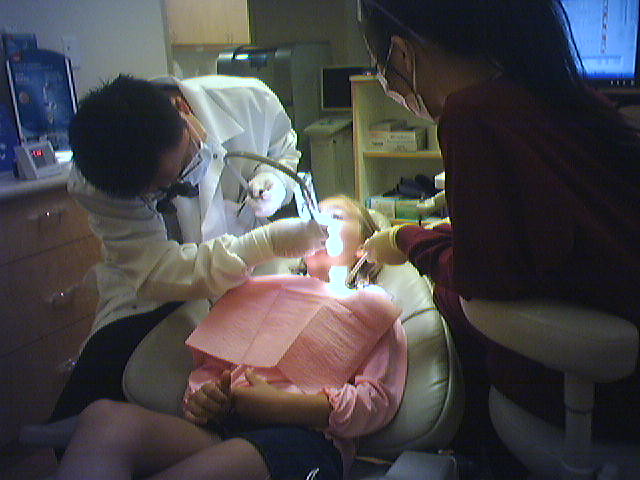In a brightly-lit dentist's office, a young girl is comfortably seated in a white leather chair, giving a thumbs up. She is dressed in a pink shirt and black shorts, with a matching pink bib around her neck to catch any splashes. The dentist, a man wearing a white coat, white gloves, and specialized glasses with magnifying lenses, is focused intently on her mouth, illuminated by a bright overhead light. To the right, a dental assistant in a burgundy shirt, white gloves, and a face mask, leans slightly forward, holding instruments and aiding the dentist. In the background, the office is equipped with brown drawers with silver handles, glove boxes, and various dental tools.